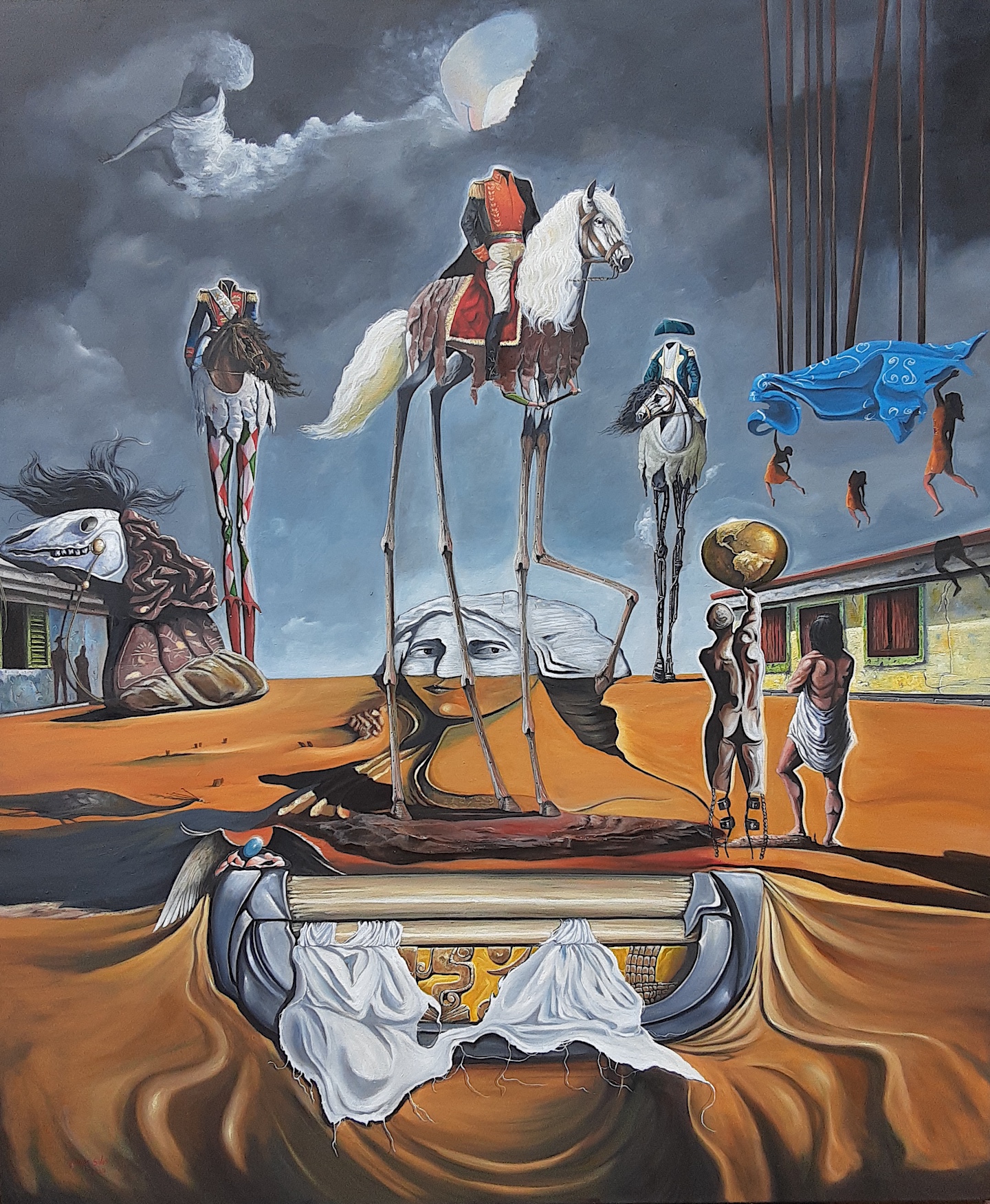The image is an abstract, Salvador Dali-inspired illustration, rich in surreal and dark elements. Dominating the scene are three headless horsemen, each seated atop horses with exaggeratedly long legs. One of these headless figures intriguingly wears a hat. The sky in the background is tumultuous, painted in varying shades of light and dark gray, suggesting a stormy atmosphere. The ground is a dark rust color, adding to the overall moody vibe of the piece. Amidst the chaos, a central figure stands out: a headless man in a red jacket on one horse. Below and to the left, there appears to be sketches of George Washington and Madonna.

The composition includes an eerie assemblage of faceless and melting figures, with one statuesque naked figure holding a golden globe. Two men stand to the right, one clutching a sphere. Deteriorated buildings with missing shutters and window glass flank the scene, contributing to its decayed ambiance. Additional surreal elements include a large skeletal horse head with hair and various draped textiles melting into the landscape. This rich tapestry of hyper-realistic and dreamlike details creates a busy, vividly colored depiction that is both haunting and captivating.